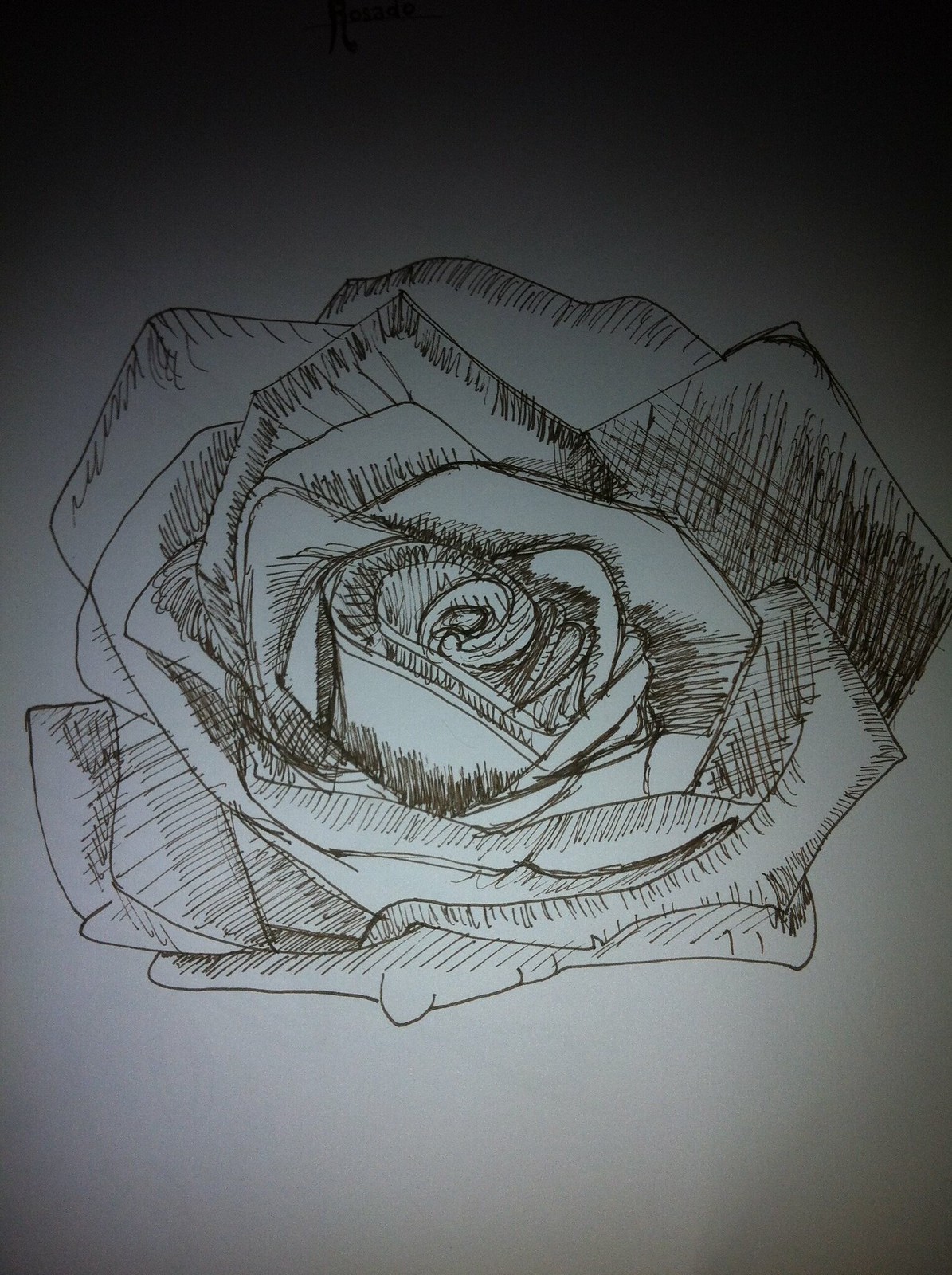This image features a meticulously detailed pen and ink sketch of a rose, centrally positioned and occupying the majority of the composition. Employing a single-width art pen, the artist has skillfully rendered the intricate, curling central portion of the rose, using precise lines and shading to distinguish the various petal shapes that unfurl in a captivating, fan-like formation. The sketch appears to be executed on white paper, though the edges of the image are darkened, possibly due to the low lighting conditions under which it was photographed. The fine lines are either black or dark gray, contrasting against the paper's light gray center, which transitions to a medium gray and ultimately to the darkened edges at the corners. The overall effect is an evocative and slightly moody portrayal of the rose, emphasizing its natural beauty and intricate structure.